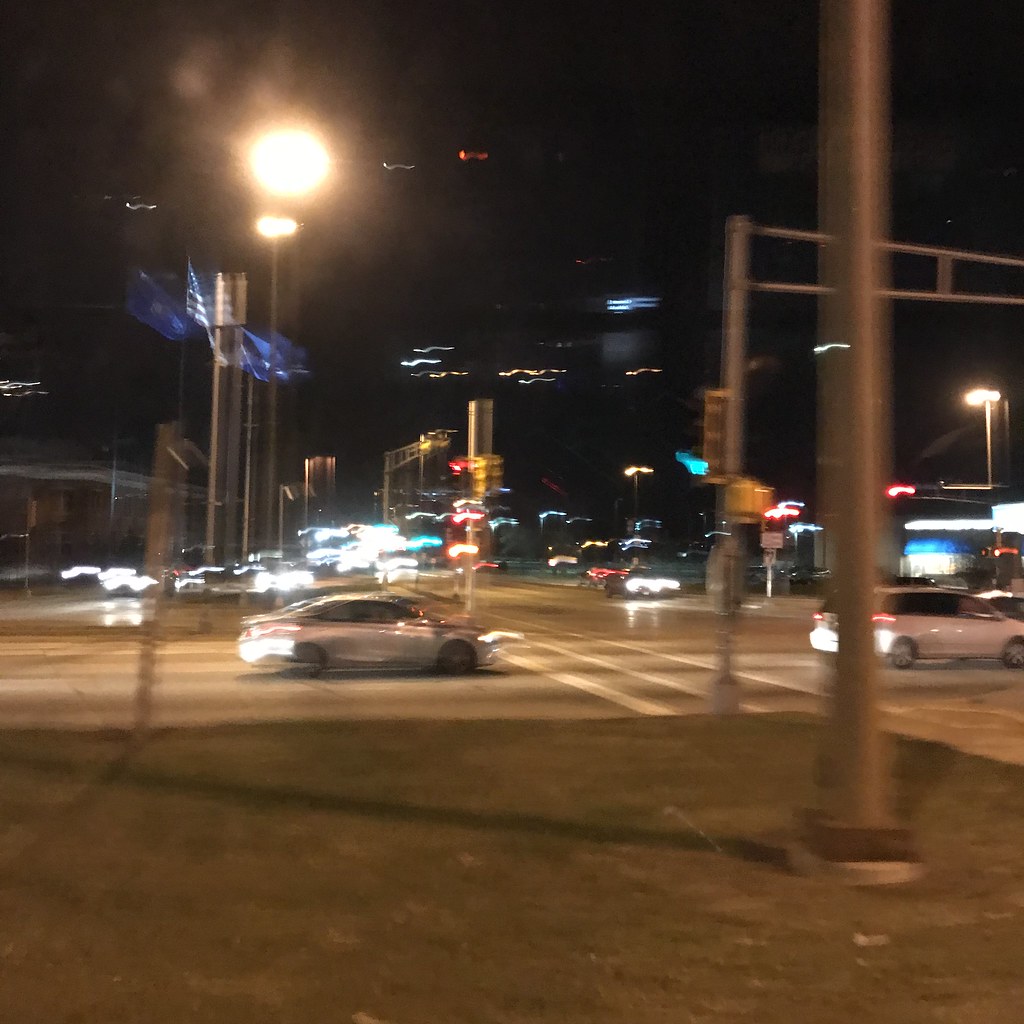This nighttime photograph captures a bustling city intersection from the perspective of a street corner. The image is somewhat blurry, suggesting the photographer may have moved the camera during the shot. In the foreground, a person stands on a patch of dead grass near several light posts. The intersection is quite busy with at least four lanes in each direction, regulated by traffic lights. A tall streetlight with an amber spotlight casts a harsh glow across the scene, creating streaks of light due to the blur.

At the intersection, a white minivan is visible in the middle, while a silver car is poised to enter. Another car is waiting patiently at the stoplight. In the distance, numerous headlights from oncoming traffic illuminate the dark background, hinting at tall buildings whose lights are visible up high. The presence of flagpoles—one bearing an American flag and the other a dark blue flag—and an ambiguous arm-like structure that resembles a railroad crossing add to the urban atmosphere. Despite the darkness, the entire scene is vividly lit by streetlights and vehicle headlights, capturing the dynamic and lively nature of the city intersection.